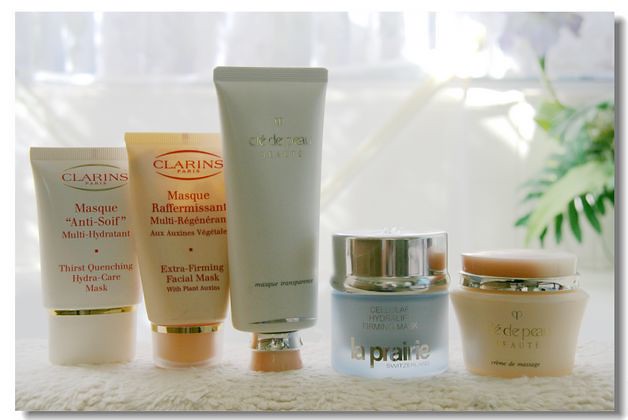In this bright and pristine photo, a carefully arranged lineup of five skincare products is set against an immaculate white backdrop, enhanced by an abundance of white light that adds to the clean and minimalistic aesthetic. The environment is exquisitely styled with white decor, making it almost monochromatic, save for a single splash of lively green provided by a palmy plant situated in the background. 

The products displayed include a range of masks and moisturizers predominantly in shades of beige and white. Among them, a mask from Clarins stands out with its descriptive labeling: "Anti-Sweat, Multi-Hydrant, Thirst Quenching, Hydro Care Mask." Another Clarins product, labeled in French, reveals itself as an "Extra Firming Facial Mask." The collection also features a taller bottle whose logo remains indistinct and another product from a brand that seems to be La Peri, although the exact spelling is uncertain. Completing the lineup is a smaller container, also without a discernible logo.

The assortment rests atop a clean, neutral mat, their neat arrangement possibly indicative of a curated skincare routine or a promotional image for a personal selection of favored products. Each item casts a subtle drop shadow, suggesting a professional studio setup, likely intended for a website showcase or a catalog. Together, these elements create a serene and luxurious scene that underscores the elegance and efficacy of the skincare products on display.